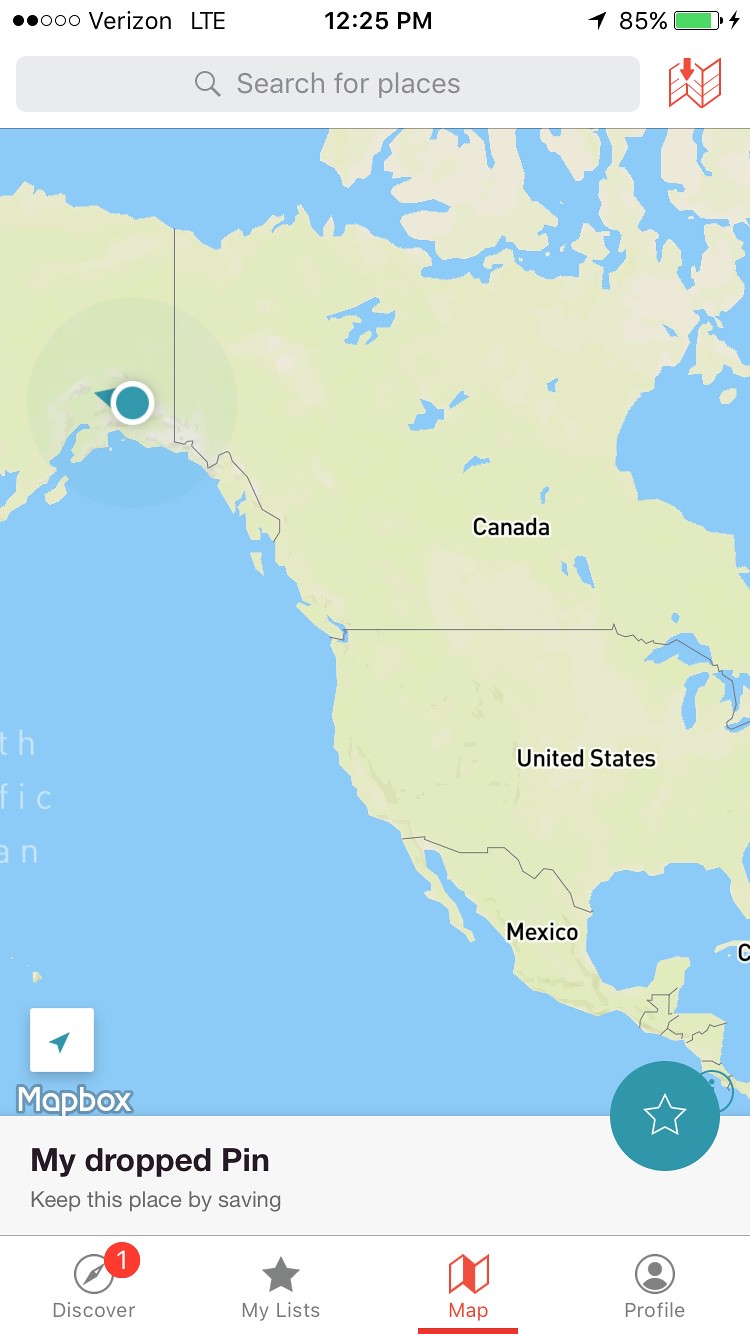The image features a detailed map interface. In the bottom left corner, the map is branded with the "Mapbox" logo. Above this logo, there's a box with an arrow pointing slightly to the right, underneath text in gray and black letters that says "My Dropped Pin - Keep this place by saving." 

Four radio buttons labeled "Discover," "My List," "Maps," and "Profile" are prominently displayed. The central portion of the image showcases a map with a blue dot positioned within the state of Alaska. The map displays geographical sections of Canada and most of the continental United States, although the eastern coast, including the tip of Florida, is partially cut off. All of Mexico is visible. Additionally, there is a circle featuring a white star on a green background.